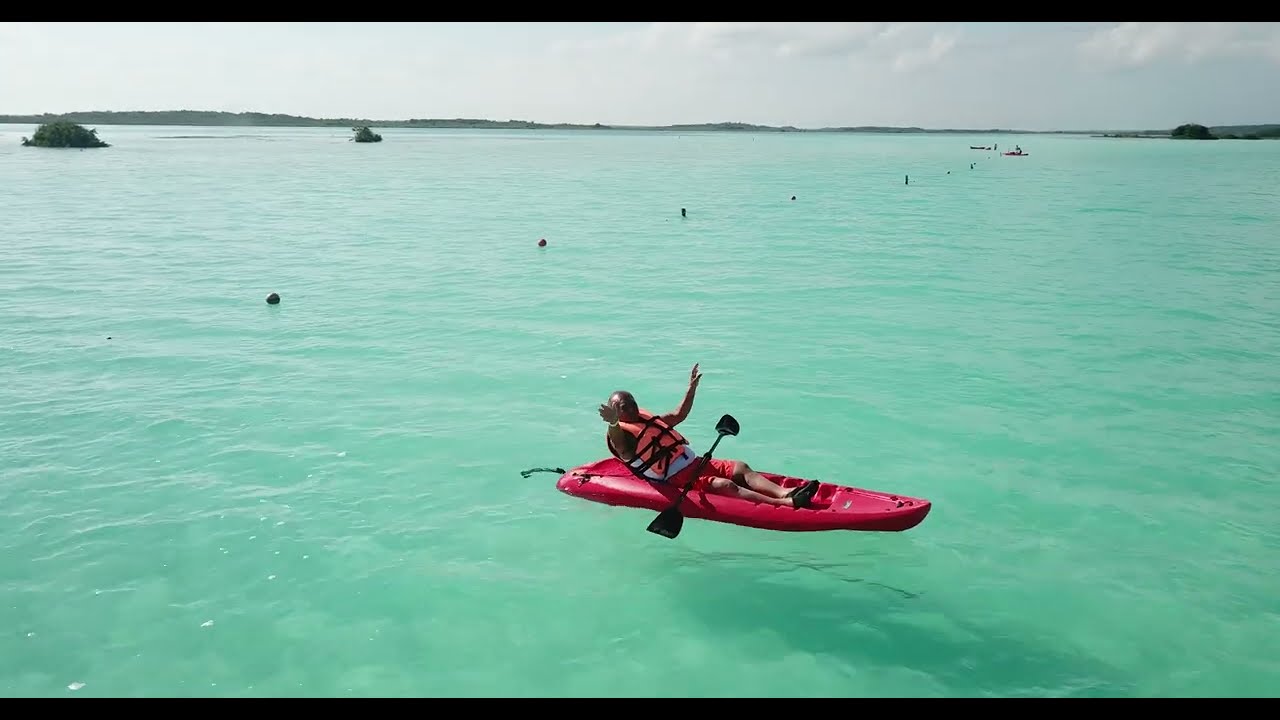In this vibrant daytime photograph, a man, likely African-American, is lounging in a red kayak on a crystal-clear, greenish-blue ocean. The subject is centrally positioned towards the bottom of the horizontal image, leaning back in his seat with his arms joyfully stretched upwards, akin to a roller-coaster pose. He wears a life jacket and rests a double-headed paddle across his lap. The clear waters dominate the image, exuding hues of aqua, light green, blue, and white.

In the background, a line of small, dark-colored buoys floats atop the ocean, and a faint silhouette of another kayaker is discernible on the distant horizon. Towards the very back, where the ocean meets the sky, outlines of several islands and landmasses, including two larger rocks on the left, are visible, under a slightly clouded blue sky. The entire scene is bathed in sunlight, casting a distinct shadow of the kayak on the shimmering water.